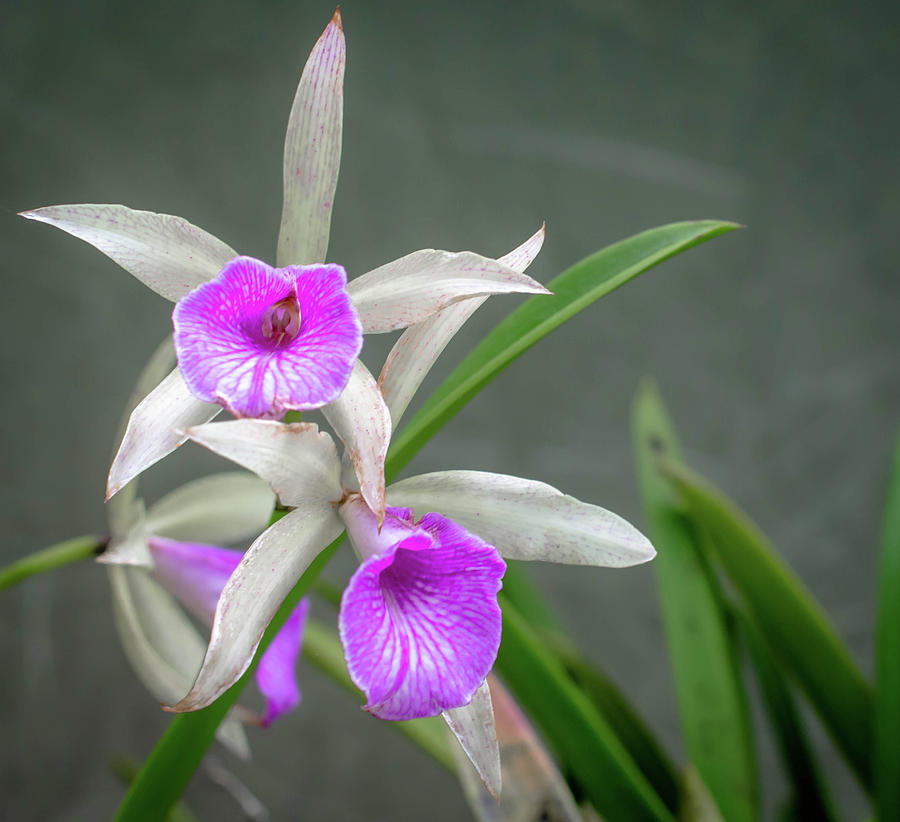This detailed photograph captures two up-close blooms of what appear to be white flowers, possibly orchids or lilies, against a gray blurred background. The prominent flower is off-center to the left and showcases five star-shaped petals, predominantly white with subtle purple striping and dots near the tips. At its heart, the flower reveals a strikingly vibrant purple center with vein-like structures and the deep, magenta-shaded throat, highlighting the stamen nestled inside. The second flower, positioned slightly behind and out of focus, mirrors the intricate beauty of the foremost blossom. In the lower right-hand corner, slender, pointed green leaves extend gracefully, possibly indicating stalks. This modern, close-up photograph beautifully emphasizes the delicate contrasts between the vivid purple and pristine white of the flowers, set against a soft, unobtrusive gray background.